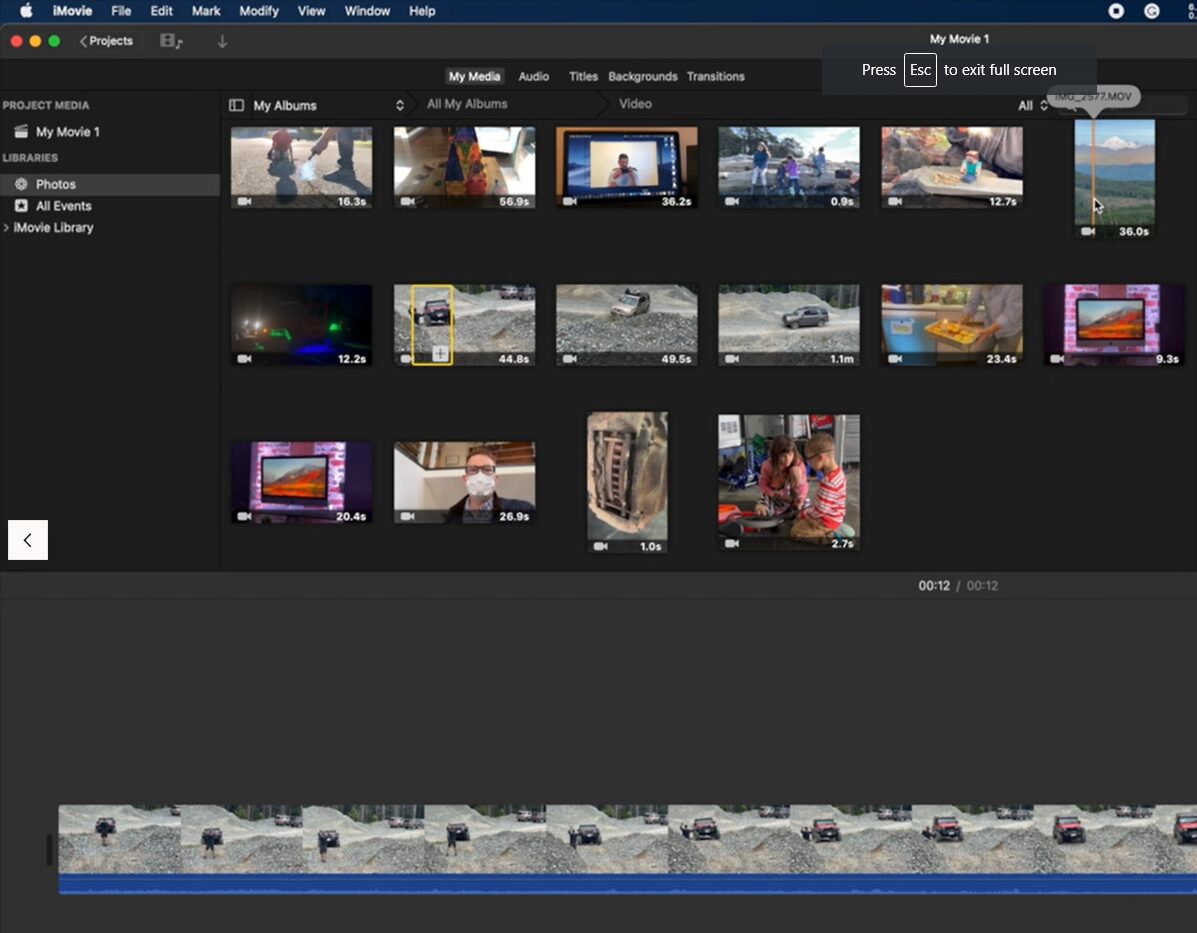The image displays the iMovie editing interface on a computer screen, with a clean, white toolbar at the top featuring options like File, Edit, Mark, Modify, View, Window, and Help. The interface also includes navigation buttons such as an 'X' to close and a refresh button. 

On the left side of the screen, there are sections labeled Projects, My Movie 1, and an instruction to press ESC to exit fullscreen mode, with a highlighted square around the ESC key. Below these sections, further categories include Project Media, My Movie 1, Libraries, Photos, All Events, and Movie Library, alongside directional arrows for navigation.

At the very top of the screen, tabs are organized into My Media, Audio, Titles, Backgrounds, Transitions, My Albums, Video, and All. The media library displays several video thumbnails. The first video appears to show a man cleaning a sidewalk, while the second one displays numerous toys. The third video thumbnail features a television screen with a man speaking. Each video thumbnail is accompanied by a time duration of 12 seconds, which is shown as "00:12/00:12" at the bottom of each video.